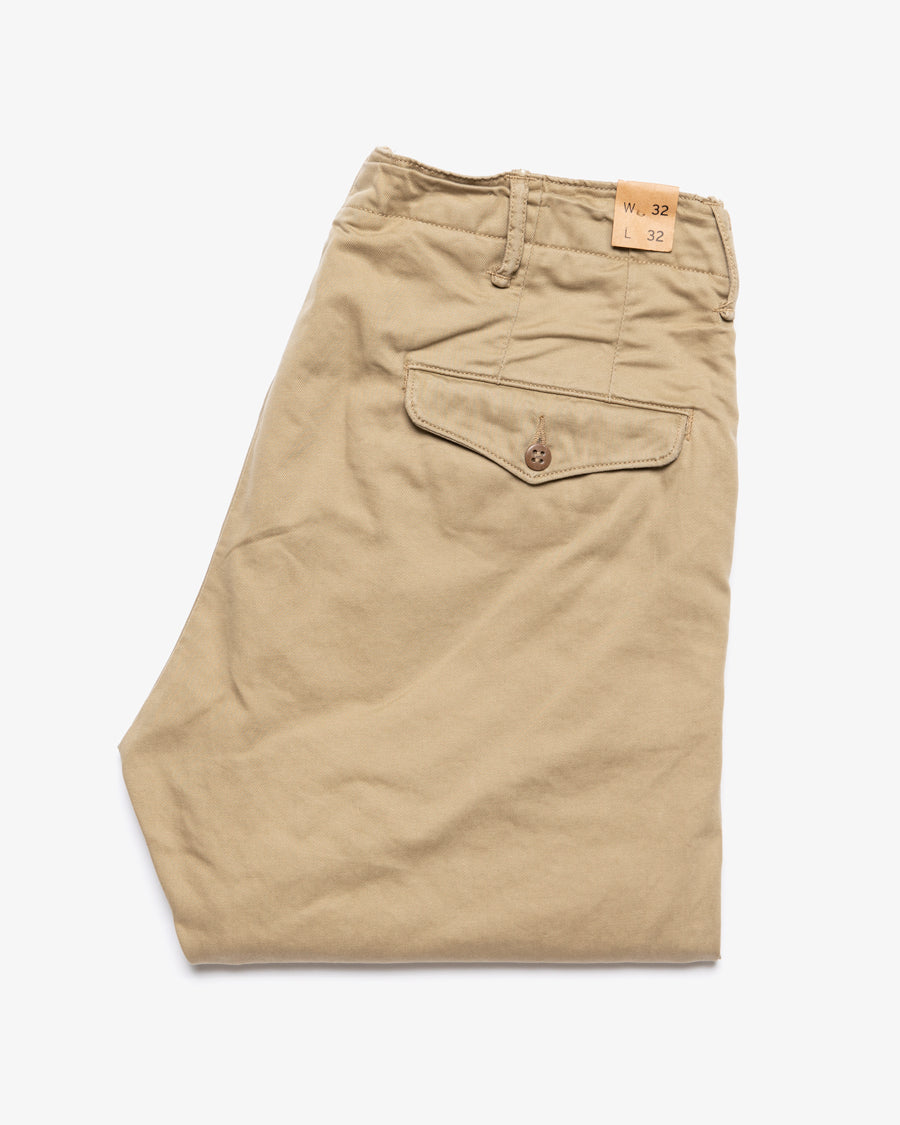The image features a pair of new khaki cargo pants, carefully folded in half and laying flat. The back half of the pants is visible, showcasing a pocket with a brown button sewn with four holes, though the seam of the pocket itself is not visible, just the flap that covers it. The pants have belts loops and exhibit notable wrinkles, indicating they may have been sitting in a pile for some time. An orange-peach colored size tag is attached at the top, specifying a waist size of 32 and a length of 32.